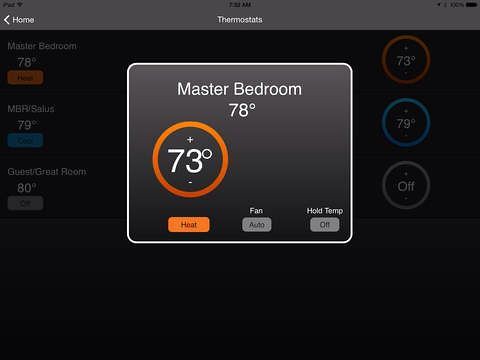This image features a high-tech thermostat with various controls and a detailed display. The thermostat itself is a sleek, black square with a light gray strip across the top, where "Home" is written in white letters accompanied by a small, left-pointing arrow. 

In the middle of the screen, the word "Thermostats" is prominently displayed in white text. Just above this, the current time "7:30 a.m." is shown in black numbers.

Central to the display is a gray square outlined in white, indicating the "Master Bedroom," where the temperature is currently 78 degrees. An orange circle within this section has a white plus sign at the top and a white minus sign at the bottom, with the temperature set to 73 degrees.

Below this temperature setting are two buttons: a red button labeled "Heat" and a gray button labeled "Auto." Above these buttons, the word "Fan" is present, alongside another gray button labeled "Off." Above these controls, the phrase "Whole Temp" appears in white text.

Background information includes additional temperature readings and room designations: "73 degrees," "79 degrees," and "Off," as well as "Master Bedroom 78," "MBR 79," and "Guest Great Room 80 degrees."